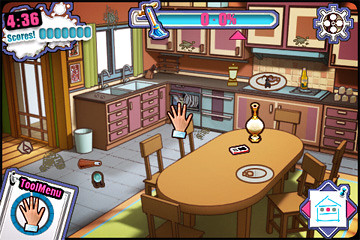This color, horizontal, rectangular image is a detailed screenshot from a child's video game, set in a kitchen. The central feature is an oval light brown kitchen table with six matching chairs, located towards the right side of the room. Adorning the table is a white and brown vase, a white and red form, and a white plate positioned on the right side. The kitchen backdrop includes brown cabinets and black countertops.

The top left corner of the image displays the time "4:36" in pink, with a teal score display featuring teal ovals and the text "scores!" Below that is a detailed percentage bar set in blue with pink text reading "0.0%" and a pink arrow beneath it. In the center of this bar is an image of a broom with a gold handle.

The bottom left corner features a board labeled "TOOLMENU" in pink, with a white background outlined in blue. Within this board is a blue circle enclosing a hand symbol. The bottom right corner showcases an icon of a house in a white square, framed by triangles on all sides—blue on the top and bottom, red on the left and right. Additionally, this corner contains two adjacent square boxes, one depicting a room with a mix of blue, grey, and pink colors.

The upper right corner displays a settings symbol represented by a seven-pointed circle with smaller circles inside, rendered in silver, brown, and white. Prominently noted within the top background is a zero of zero progress statement. The kitchen space also includes various fixtures such as a stove, a sink, and additional mounted cabinets, contributing to the room’s busy, utilitarian appearance.